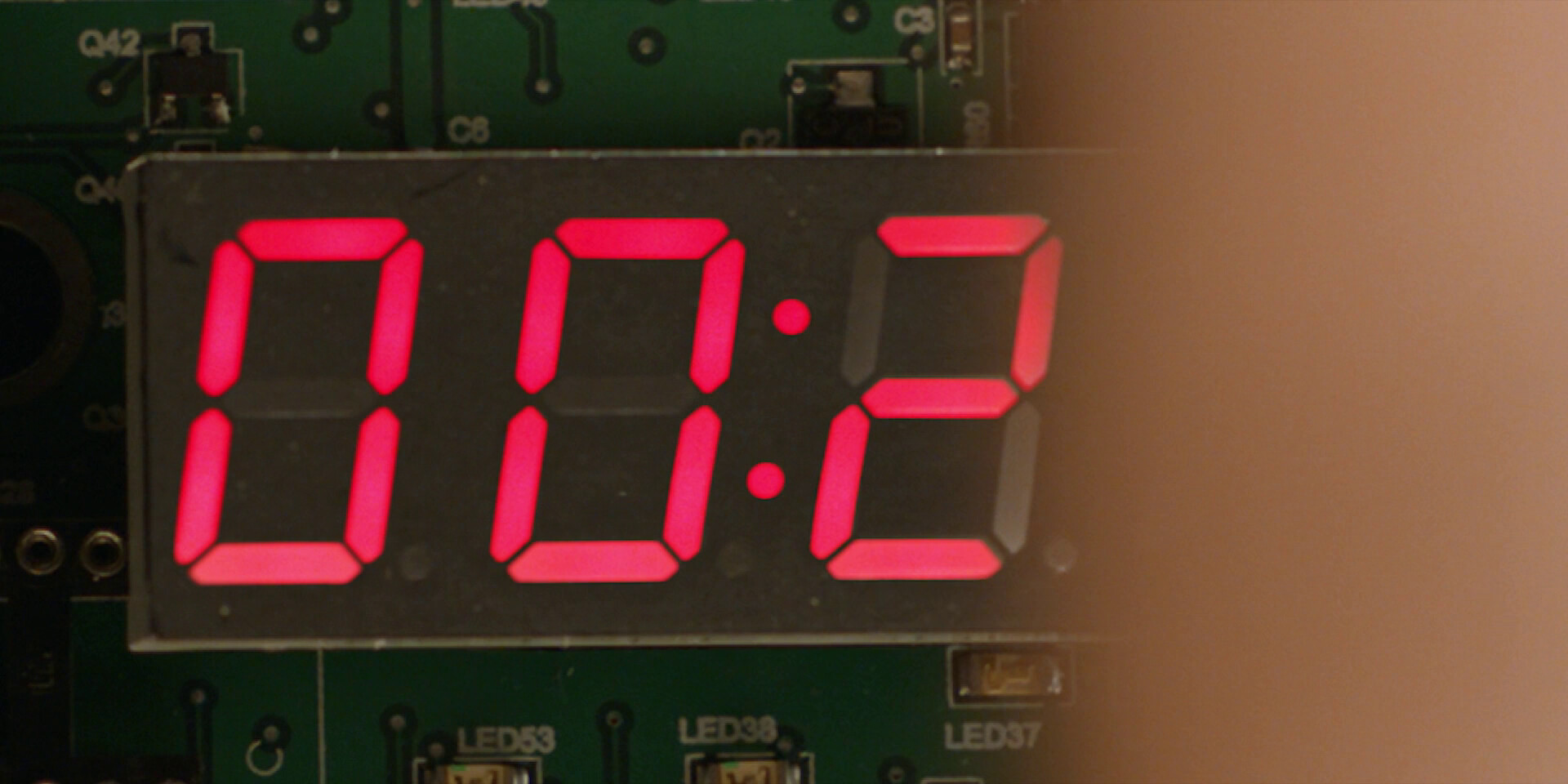A close-up photograph captures a rectangular digital clock, reminiscent of those seen in suspenseful scenarios, perhaps even resembling a bomb timer. The clock currently displays "00.2" in bright red digits. However, the full display is partially obscured by a thumb or a finger, adding a sense of human interaction or obstruction to the scene. Surrounding the digital clock are several green control panels adorned with intricate patterns reminiscent of computer circuitry. Scattered across these panels are small letters and numbers, such as "Q42," "C8," and "LED53," presented in white writing. The combination of the digital clock and the detailed control panels creates an intriguing and somewhat enigmatic composition.